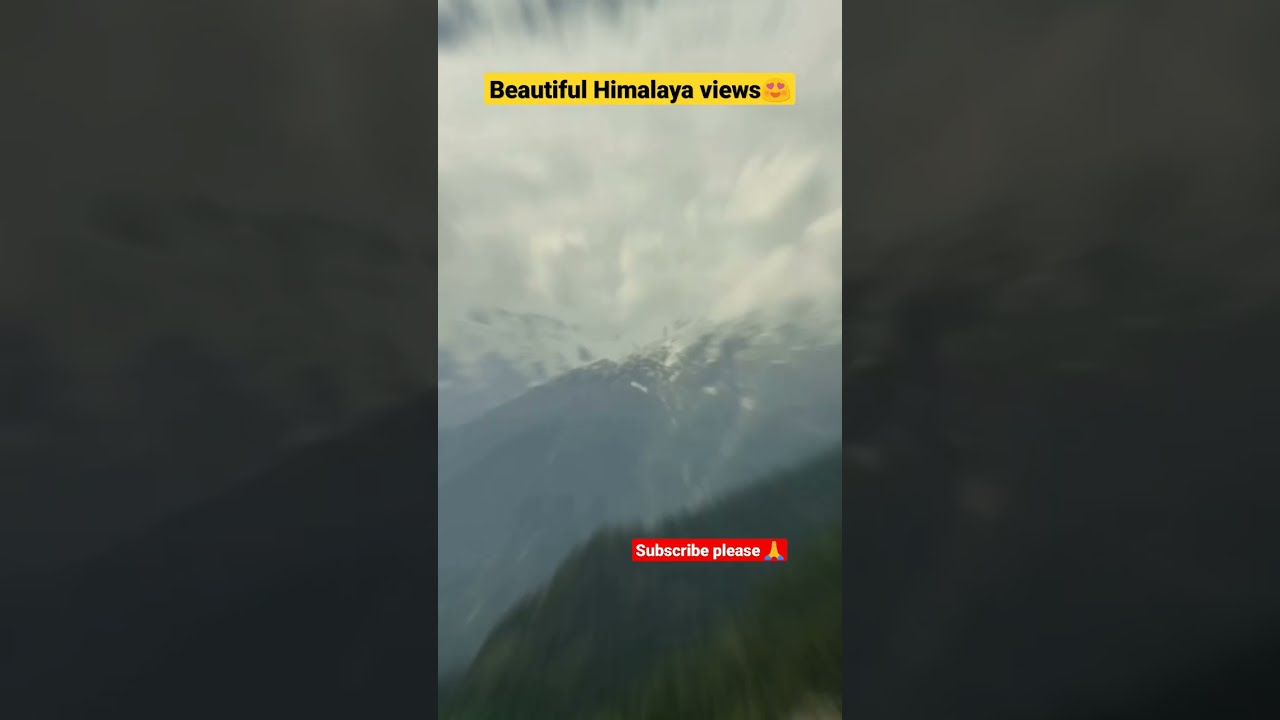The image depicts a vertical cell phone-style picture centered against a faded, zoomed-in background of the same scene. The main image showcases a stunning view of mountain ranges, where the front ridge appears lush and green but slightly out of focus, while the distant back ridge is shrouded in haze, making it hard to discern if it is vegetated. The sky takes up about half of the frame, filled mostly with clouds, some of which descend below the peaks.

At the top of the image, a yellow rectangle contains black text that reads "Beautiful Himalayan Views" accompanied by a heart eyes emoji. In the bottom right corner, a red rectangle with white text says "Subscribe Please," along with a praying hands emoji. The sides of the image display a zoomed and tinted version of the primary photo, allowing only portions of the mountain peaks to be visible. The overall effect is reminiscent of a motion blur, as if flying over the mountaintops.